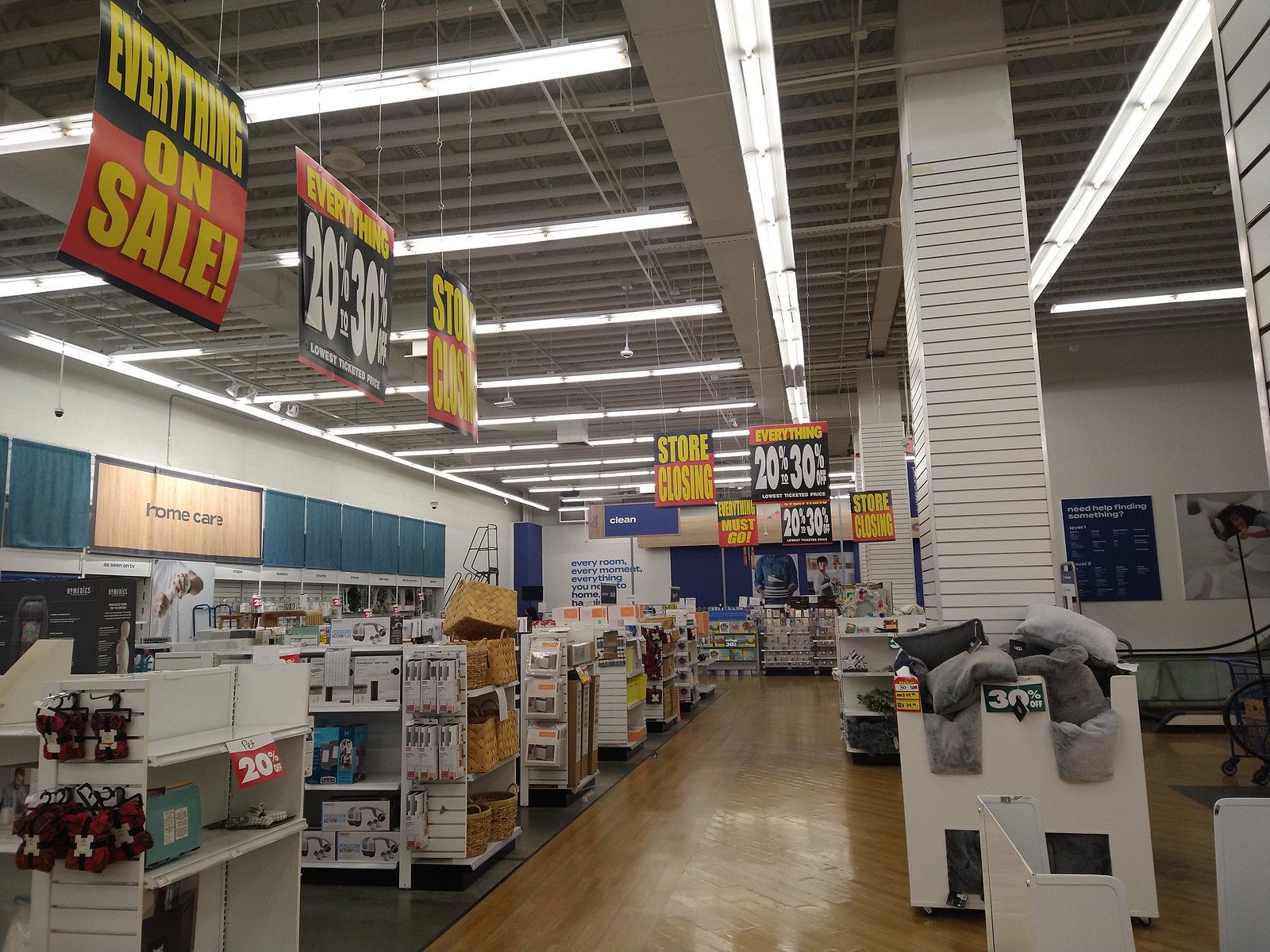This photograph captures the interior of a department store, possibly a Bed, Bath & Beyond, slightly wider than it is tall. The focal point is an aisle with a brown wooden floor, flanked by numerous white shelves stocked with various home care items such as baskets, sheets, pillows, and home electronics. To the left, a wall prominently features a sign reading "Home Care" with a wooden background and black lettering, adorned with teal squares arranged horizontally. The industrial, exposed ceiling hosts long, rectangular hanging lights, with numerous sale signs suspended from them. These signs, in black, red, and white, loudly proclaim "Store Closing" and "Everything 20-30% Off." The far wall boasts five such signs, while the left wall has three. In the bottom right of the image, a white cardboard box filled with pillows, priced at 30% off, is visible. The far end of the aisle is somewhat blurry, making it difficult to discern specific details beyond this point.